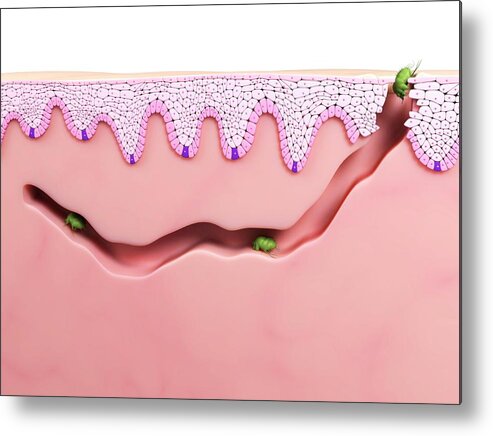This artwork intricately depicts the infiltration of parasites below the surface of human skin. The side profile illustration reveals different layers of the skin, starting with a wavy pink epidermis layer at the top, followed by a bubbly, white layer underneath. The skin cells are clearly delineated, resembling a typical human skin diagram. Instead of hair follicles, the image showcases three green bug-like creatures, which appear similar to fleas or beetles. These parasites have burrowed tunnels through the layers, analogous to ant tunnels in the ground. One of the bugs is seen deeply embedded in the skin, another midway, and the last one just starting to enter, traversing past the white bubbly area into the deeper layers. This visual serves a detailed representation of the burrowing behavior of skin parasites and their journey below the skin's surface.